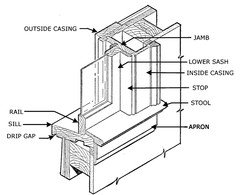The diagram, presented on a white background, is a detailed black-and-white cross section of a window. Labeled parts include outside casing, jam, lower sash, inside casing, stop, stool, apron, rail, sill, and drip gap. Each component is clearly marked with black arrows pointing to the respective parts of the window structure, showcasing how different pieces of wood fit together. The schematic delineates various sections such as the outside and inside casing, the lower sash, and additional elements like the stop, stool, and apron, all integral to the window assembly. Despite the absence of color, the comprehensive labeling provides a clear understanding of the construction and arrangement of the window components.